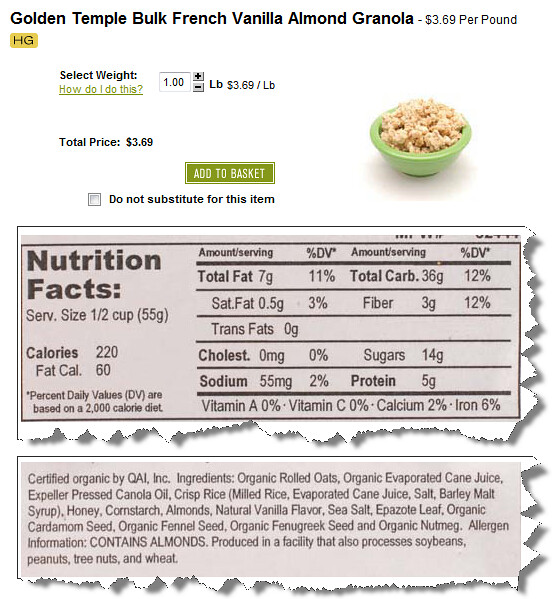The image displays a detailed online shopping cart interface for a product. At the top, "Golden Temple Bulk Vanilla Almond Granola" is prominently listed, priced at $3.69 per pound in black text. The label "HG" is positioned just below the product name. Beneath this, there is an option to select the weight, starting at 1.00 pounds, with plus and minus signs to adjust the quantity as needed. The total price of $3.69 is displayed, and an "Add to Basket" button with a green background and white text is available. There's also an option to check or uncheck a box labeled "Do not substitute for this item."

On the right side of the shopping cart interface, a green bowl containing brown granola ingredients is depicted. Below this image, a nutrition facts label and an ingredient list are presented in gray, with black lettering for readability.